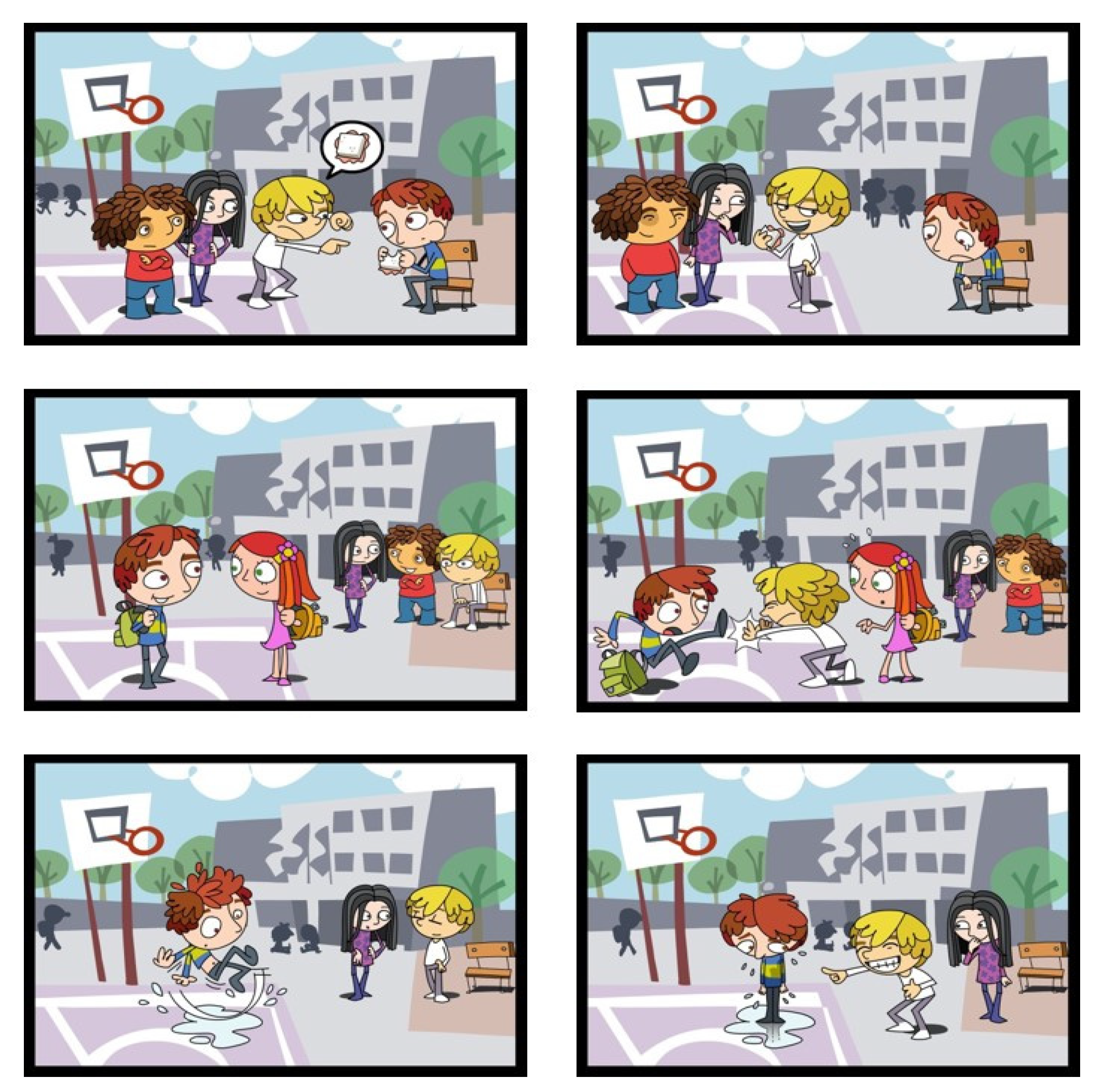The image is a six-panel comic strip depicting a playground scene on a basketball court with four children. In the first panel on the top left, three kids—two boys and a girl—are interacting. One of the boys, wearing a white shirt, is pointing to another boy in a striped shirt who is sitting on a bench eating a sandwich. The second panel shows the boy in the white shirt taking the sandwich from the boy in the striped shirt, who begins to cry. The third panel shows the boy in the striped shirt talking to a girl who has newly entered the scene. In the fourth panel, the boy in the white shirt pushes the boy in the striped shirt, causing him to slip on a puddle of water. In the fifth panel, only three of the children are visible, focusing on the aftermath of the scuffle. Finally, the bottom right panel shows the bullies— the boy in the white shirt and the girl in the purple shirt—laughing at the boy in the striped shirt, who is now wet from slipping. This comic illustrates a series of bullying incidents, escalating from teasing to physical aggression.